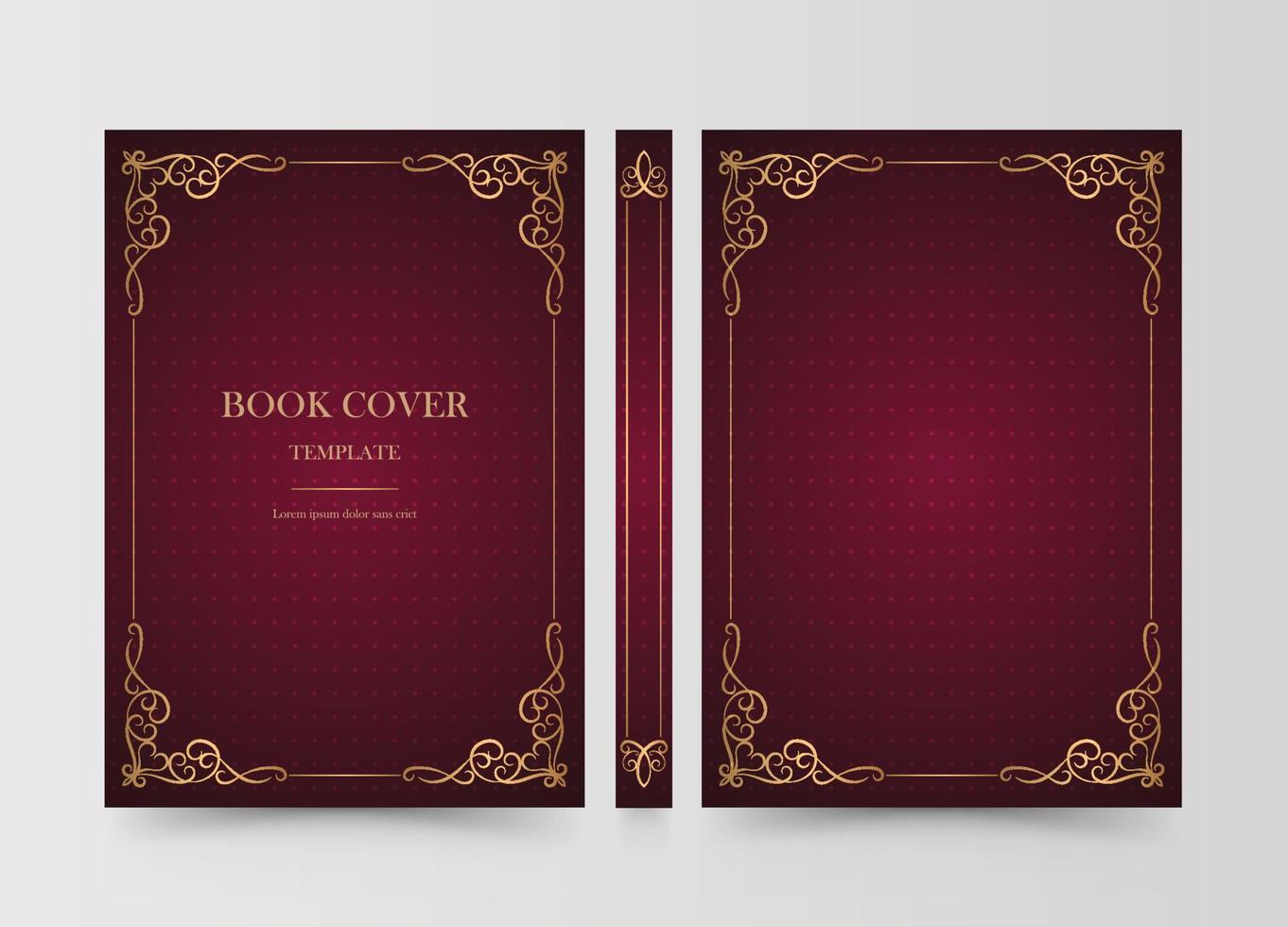The image depicts a meticulously designed book cover template set against a very light gray background. The book cover, presented in a landscape orientation, features a rich maroon or burgundy color and is adorned with intricate gold ornate designs in the corners that connect around the edges with fine gold lines, creating a cohesive elegant border. The front cover prominently displays the words "Book Cover Template" in large gold letters, with smaller text underneath featuring placeholder text in Greek or Latin, possibly "lorem ipsum." Both the front and back covers share similar ornate edging with a Celtic swirl design, enhancing the luxurious appearance. The spine of the book, also maroon, carries the same gold ornate edging on the top and bottom, maintaining the sophisticated aesthetic. The overall effect is one of elegance and artistic flair, showcasing a professional and visually appealing book cover template.